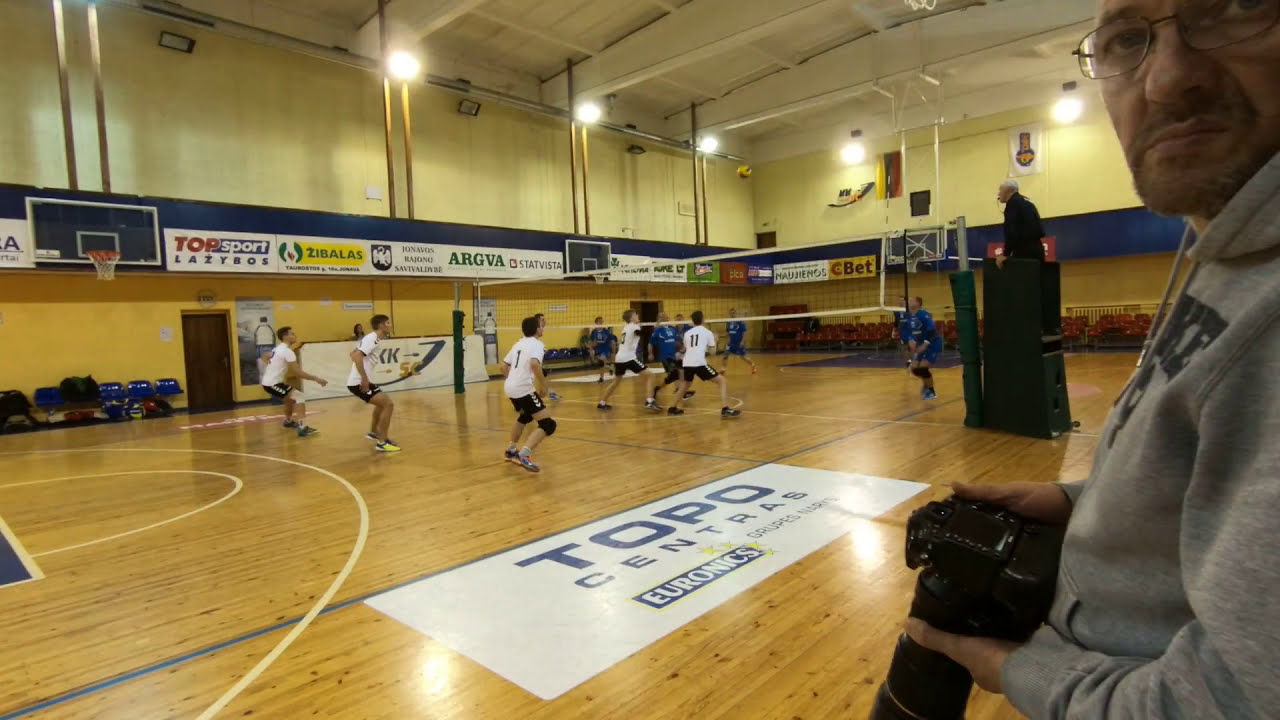This detailed image captures an indoor men's volleyball game taking place in a gymnasium or auditorium. The court, made of light, glossy wooden panels with a yellowish-brown hue, spans the bottom half of the photo and features a prominent white logo that reads "Topo Centros Euronics" in blue font, positioned diagonally. The walls of the room are primarily light yellow, with blue-striped white banners circling the space, contributing to the bright ambiance. Above, the white metal ceiling is outfitted with lights.

The image is captured from a slightly slanted perspective, revealing both teams in action: one in white jerseys and the other in blue. Players are equipped with knee pads and sneakers, indicative of a high-energy match. A referee, clad in black, is seated in an elevated black perch next to the volleyball net, which is centrally placed. On the right side, the nearest object is a photographer with a goatee, glasses, and a gray hoodie, holding a camera.

Additionally, there are some blue chairs set up along the wall, possibly for spectators or team members. Basketball hoops mounted around the court suggest multi-sport use. The partition and balcony area feature darker blue accents contrasting with the light yellow walls, while sturdy dark-colored pillars add to the structural integrity of the spacious venue.